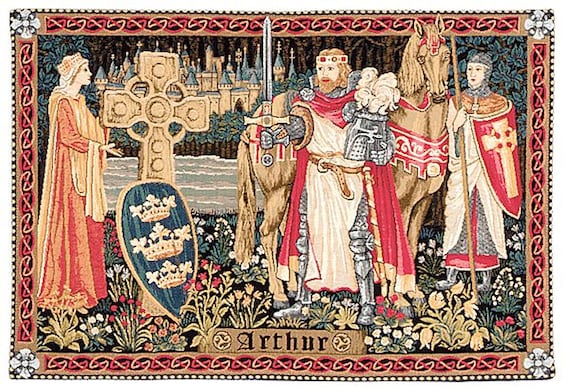This detailed photograph captures a medieval-themed tapestry depicting King Arthur. At the bottom of the tapestry, the name "Arthur" is stitched in black text against an ornate gold background. The border of the tapestry is an intricate design of red and white lines, featuring white flower patterns in each corner.

At the center, the regal King Arthur stands facing left, wearing a red cape over light tan robes and armor. He holds an ornate sword vertically in one hand, and in the other hand, he holds his silver helmet along with an ornate headpiece representing a crown. To his right stands a brown horse, adorned with a sash, being held in place by another knight. This knight, dressed in silver armor, a white robe, and a red cape, carries a large red shield emblazoned with a cross.

To the left of King Arthur, a large stone crucifix with a blue shield featuring a crown motif rests on the ground. A woman in a light and dark orange robe stands beside the crucifix, crowned and gazing towards the knights. In the background, a castle and flowers add to the tapestry's rich, historical ambiance.